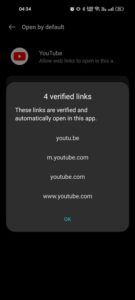**Descriptive Caption:**

A blurry screenshot of a cell phone screen displaying a YouTube-related web page. At the top of the image, the screen shows an array of typical status icons, partially readable "414," and tiny symbols that are normally present on a cell phone. Below this, the header indicates "open by default" with an arrow pointing to the left. The familiar red and white YouTube logo appears to the left with the word "YouTube" written next to it.

Just beneath, a sentence starts with the word "allow," but its rest is illegible due to the blurriness and small font size. A light gray box underneath highlights "4 verified links," with the description "These links are verified and automatically open in this app." The verified links listed include "Y-O-U-T-U.B-E," "m.youtube.com," "youtube.com," and "www.youtube.com." A green circular tab with "OK" on it appears at the bottom of this section.

This text aims to inform users about verified YouTube links to prevent them from clicking potentially misleading or unsafe links. The background of the screen is predominantly black with a central dark gray square containing white text. No other text or visual details are present in the screenshot.